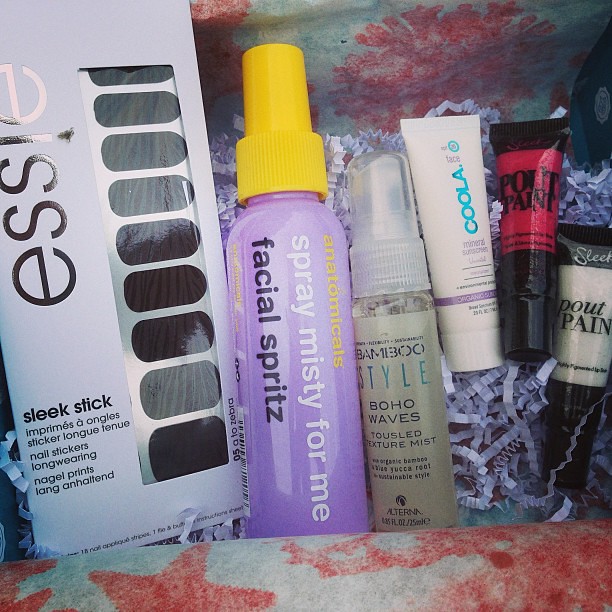The image displays an artfully arranged gift box filled with an assortment of toiletries and beauty essentials. The box is lined with light blue gift wrap adorned with red designs, including snowflakes and stars, and padded with purple crinkle cut paper for cushioning. From left to right, the items featured in the box are:

1. **Essie Sleek Stick Press-on Nails** – A sleek stick product from the brand Essie, ideal for an elegant manicure.
2. **Facial Spritz** – A prominent purple bottle with a yellow twist-off cap, intended for a refreshing facial mist.
3. **Bamboo Style Boho Waves Texture Mist** – A small bottle labeled "Bamboo Style Boho Waves Tau Silt Texture Mist," enhancing hair texture.
4. **Kula Face Cream** – A petite white container likely containing moisturizing cream.
5. **Sleek Pout Paint** – Two small containers labeled "Sleek Pout Paint," one in pink and the other in white sheer.

The coherent and thematic arrangement suggests this is a thoughtfully curated gift set, perfect for pampering and beauty routines.